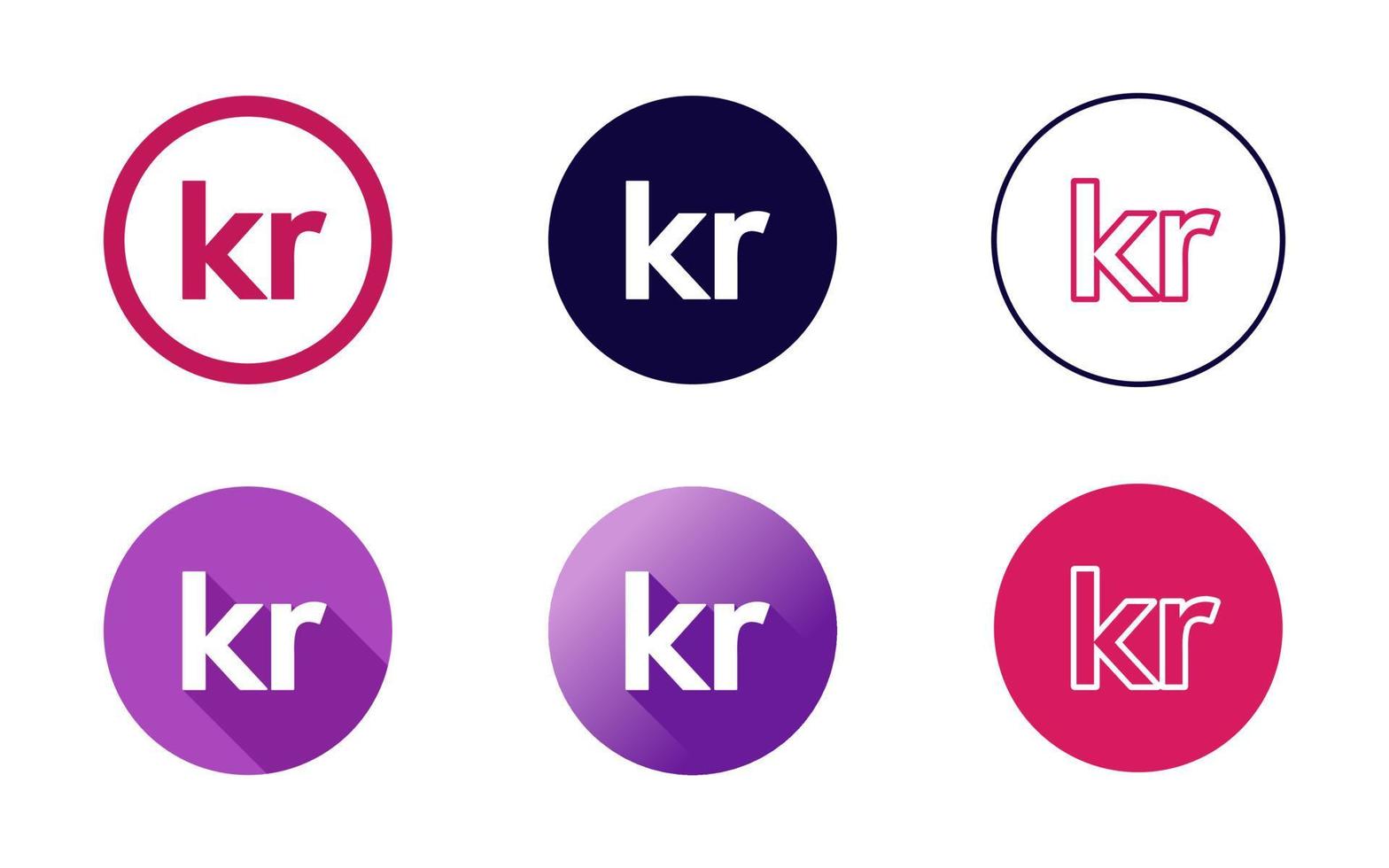This image showcases a comp sheet for a logo of a company called KR, featuring six circular logo designs, each with the lowercase letters "kr" centrally placed. The logos are arranged in two rows of three. 

1. The upper left logo features a circle with a red (or magenta) ring and white interior, holding red text for "kr".
2. To its right, the second logo presents a solid black circle filled with white text for "kr".
3. The third logo in the top row depicts a white circle outlined in black with "kr" in white, outlined in red (or possibly purplish-red).
4. The bottom left logo contains a completely filled purple (or purple-pink) circle with white "kr" text, which casts a shadow to the bottom right, giving it a 3D effect.
5. In the middle of the bottom row, the logo shows a purple gradient circle, with shading that makes it appear almost spherical, featuring white "kr" text also casting a shadow.
6. The final logo on the bottom right displays a completely filled red circle with "kr" in red, outlined in white.

These varied designs provide different stylistic options for the client to choose from, each emphasizing different color palettes and design elements.